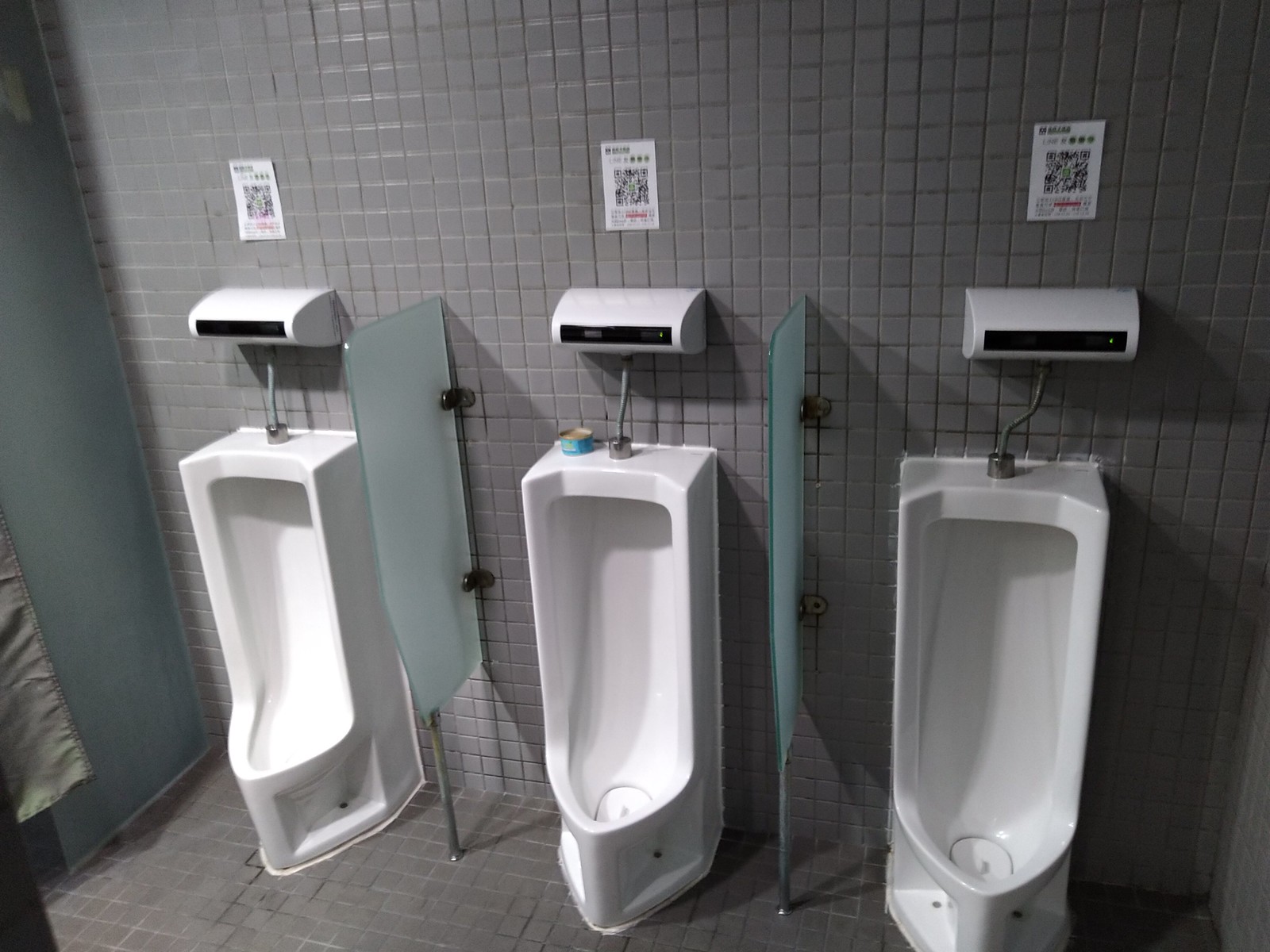The photograph captures a gray-tiled public restroom featuring three white, floor-to-ceiling urinals in a row. Centered along the left side of the image, a partial bluish wall can be observed. Each urinal is separated by frosted glass partitions and equipped with a sensor system, indicating they are automatic flushers. Above each urinal's sensor, a piece of paper displaying a QR code is affixed to the wall. Notably, the middle urinal has a small blue can, likely an air freshener, placed on it. Both the gray walls and the floor are covered with identical small square tiles, contributing to a uniform aesthetic.